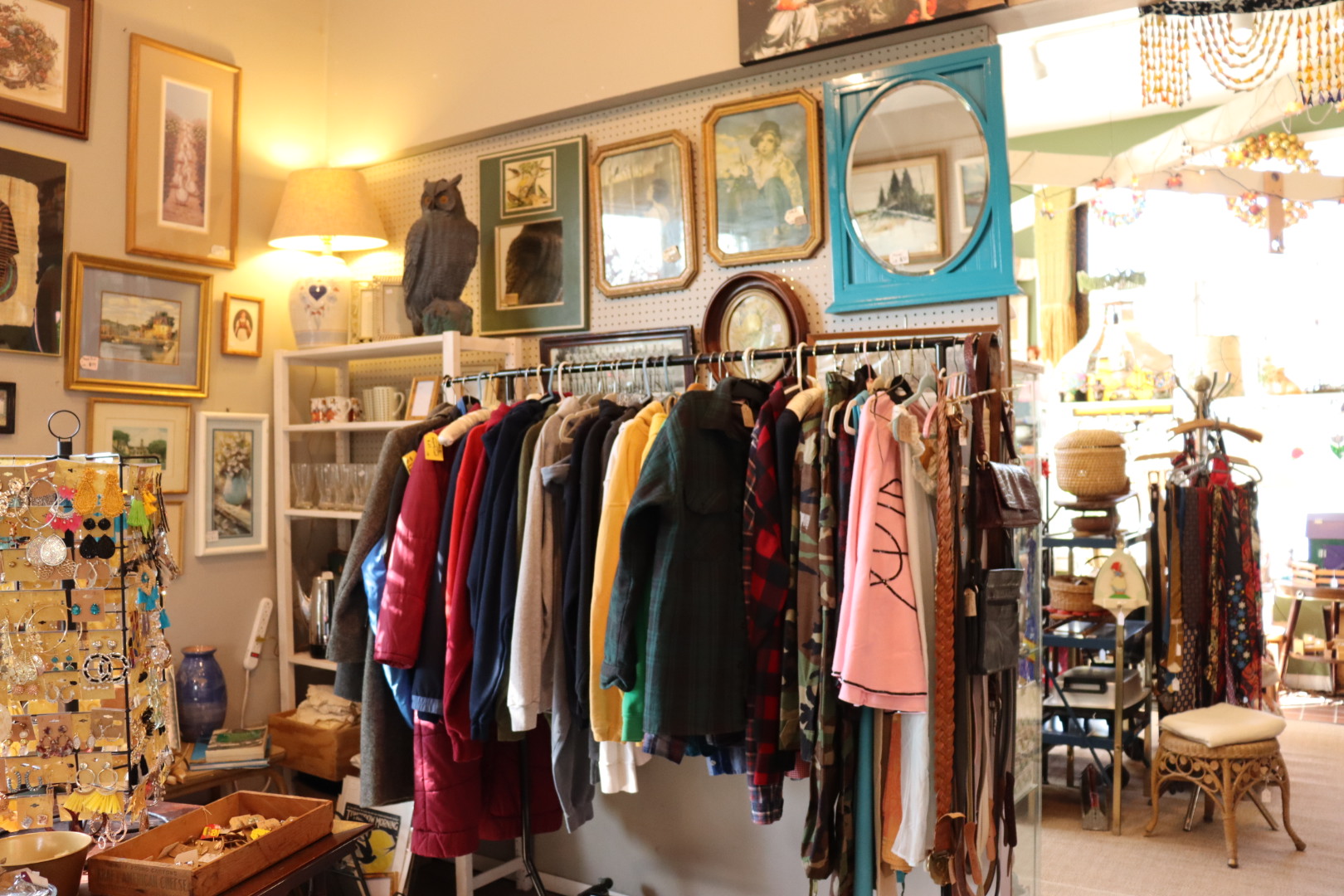The image depicts the interior of a quaint, almost antique-looking thrift or secondhand store. Central to the photograph is a clothing rack bursting with a colorful assortment of women's clothing in reds, blues, yellows, greens, and pinks. Behind this, a corkboard wall adorned with mounted mirrors and framed paintings, including landscapes—possibly one of a road in San Francisco—sets a nostalgic background. To the left, more framed paintings are displayed, alongside a white shelf holding various glassware and kitchen items, topped with a stone owl statue and a country-style lamp.

In the foreground, a table showcases a wooden box filled with trinkets and a spinning rack displaying women's earrings. The entryway to another room is embellished with hanging beads and reveals more racks filled with scarves, baskets, and other items. A white upholstered footstool and several smaller shelves with vases and glassware populate this second area, providing an eclectic mix of objects for customers to peruse. The walls are beige, adding to the cozy atmosphere, with some rope-like patterned artwork hanging from the ceiling. The entire space exudes a charming, filled-to-the-brim consignment shop vibe.